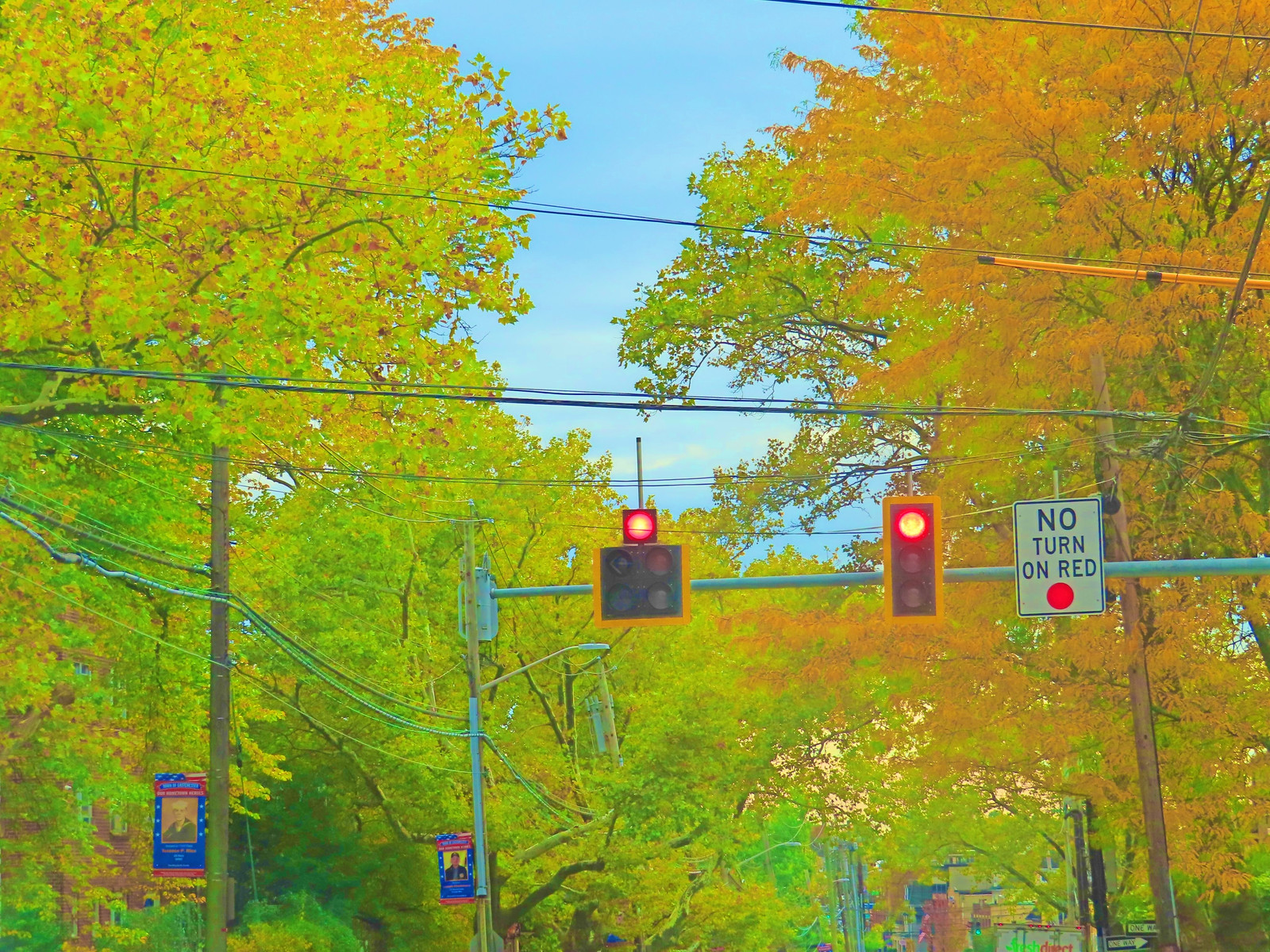The image depicts a vivid outdoor scene captured from the ground, looking slightly upward. Dominating the background is a spacious green area with clusters of trees displaying vibrant fall colors, ranging from green to bright yellow and orange. The blue sky peeks through the foliage. Crisscrossing power lines extend horizontally across the image, suspending multiple traffic lights and utility poles. Prominently featured in the scene is a horizontal green bar extending from the right side to the middle, supporting a rectangular traffic light with a lit red signal at the top. An adjacent square traffic light with an illuminated red signal and a “No Turn on Red” sign, featuring a red dot, further emphasize the stop directive. The overall scene is highly saturated, enhancing the strikingly bright colors of the trees and surroundings.